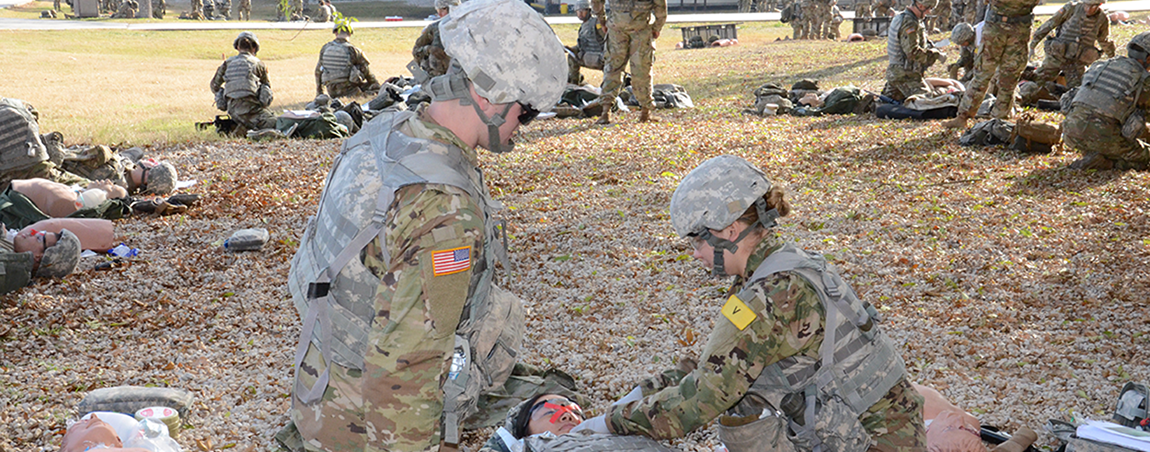This is a color photograph capturing a US Army training exercise where service members are practicing first aid on a grassy field. In the foreground, two soldiers are highlighted. The soldier on the left is a man wearing camouflage with a protective vest, helmet, and sunglasses, sporting an American flag patch on his shoulder. He is kneeling upright. To his right is a woman also in camouflage, wearing glasses, and identified by a yellow patch with the letter V on her shoulder. She is kneeling towards the ground, tending to a man lying on the ground with red tape marked on his face. Surrounding them are cloths, first aid equipment, and various training materials. The immediate background reveals other similar groups of soldiers practicing first aid on either test dummies or fellow soldiers, each group engaged in their own training session. In the far background, more military personnel and possible instructors are visible, standing or sitting in the field, with some appearing to look off into the distance. The wide image captures a sizeable grassy area with scattered leaves, leading up to a road visible towards the horizon, emphasizing the outdoor, comprehensive training environment.